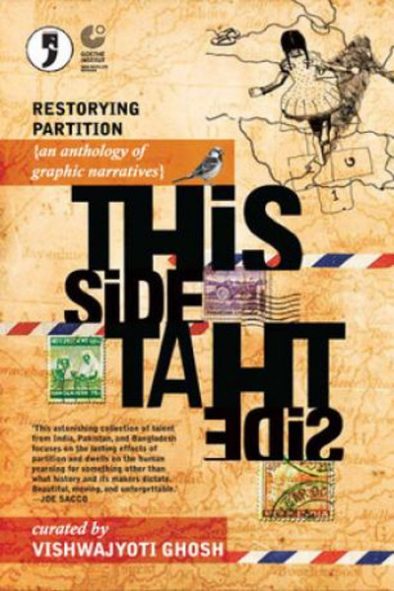The image appears to be the front cover of a book styled poster, primarily featuring a collaged, tan, and orangish-beige background that resembles an old, possibly treasure, map. Dominating the cover at the top is a drawing of a girl in a dress walking across the map, positioned at the upper right. The title "Restorying Partition" is prominently displayed to her left. Below this title, a horizontal orange bar contains the phrase "An Anthology of Graphic Narratives," accompanied by a small bird perched beside the text. Centered on the cover in bold black letters is the title "This Side, That Side," with some letters creatively reversed, giving it a unique touch. The cover is visually occupied with several old, used-looking stamps in green, purple, and orange scattered around, some positioned towards the image's middle, left, and bottom. A black paragraph is barely readable above another orange bar at the bottom right of the cover. The orange bar itself bears the text "Curated by Vishwajyoti Ghosh" in white. Additional decorative elements include three red, white, and blue barber pole-like strips on various parts of the cover and a circular emblem with a black apostrophe inside it at the upper left. The overall composition is rich with detailed text and imagery, blending multiple colors including tan, brown, red, white, blue, green, and black, creating an intricate and somewhat cluttered but captivating collage-like appearance.